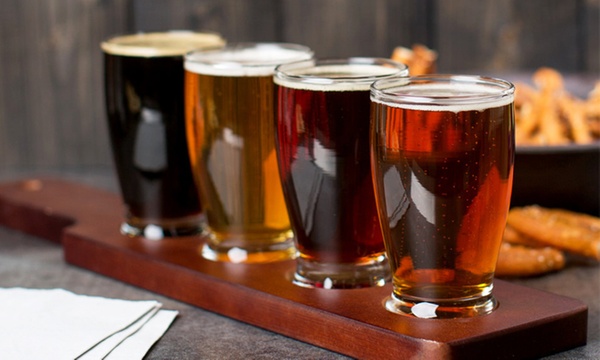This detailed indoor photograph captures a close-up of four glasses of beer arranged diagonally on a rectangular wooden serving tray, which features circular openings to securely hold the glasses. The tray is set upon a grayish-black, stone-textured table. Starting from the left side of the image, the first beer is a deep brownish-black color with golden froth. Next to it is a lighter brown beer, followed by a maroon-colored beer, and finally, a reddish lighter-colored beer. All glasses have bits of foam at the top, indicating their freshly poured status. In the blurry background, there’s a bowl of food, likely containing fries and possibly chicken wings. Additionally, the lower left corner of the image shows the edges of three white napkins. The background wall is made of grayish-black wood, adding to the rustic indoor ambiance of the scene.